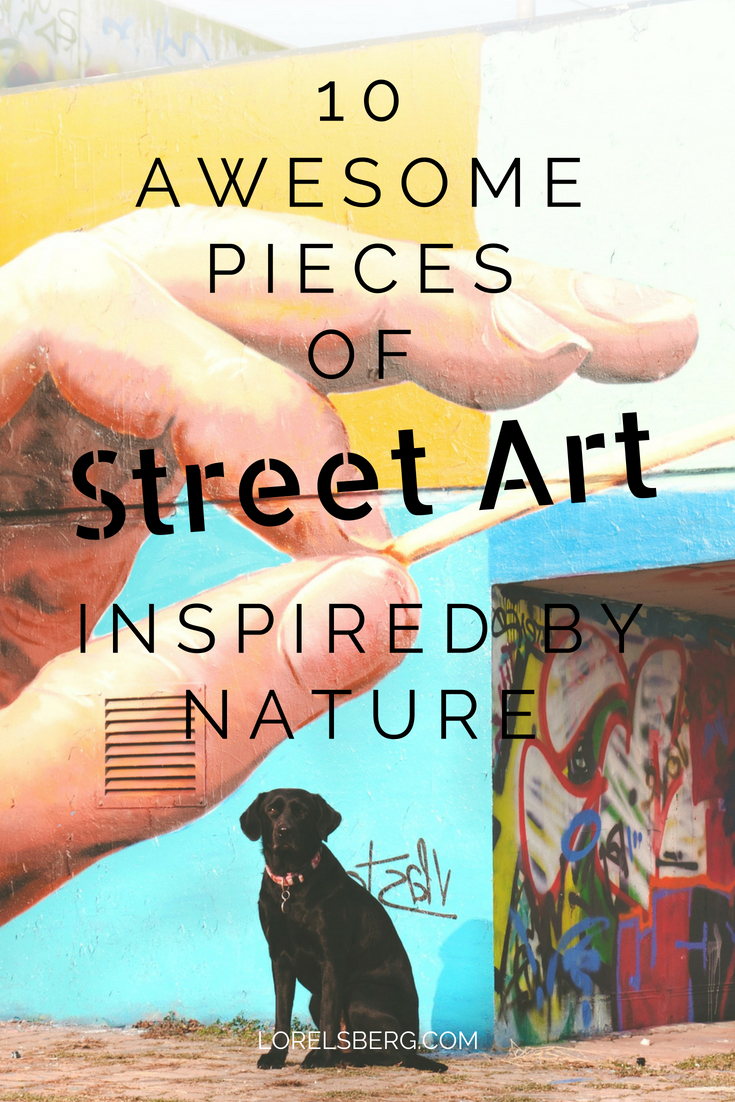This book cover vividly showcases a captivating image of a black Labrador sitting on an overgrown concrete ground in front of a graffiti-adorned wall. The wall, divided into four distinct quadrants, features a vibrant array of colors: yellow at the top left, white at the top right, light blue at the bottom left, and a darker blue at the bottom right. Dominating this artistic backdrop is a Caucasian hand, spanning across the upper two quadrants and part of the bottom left, clutching a matchstick. Above the dog and hand, black stencil-like text announces the title "10 Awesome Pieces of Street Art Inspired by Nature." The wall behind the seated dog further displays a graffiti signature, amplifying the urban aesthetic. Just beneath this primary scene, a passageway continues through the concrete structure, revealing more multicolored graffiti in hues of red, yellow, white, and green. At the very bottom of the book cover, in crisp white text, reads "loresberg.com," completing the eclectic and visually rich design that immerses viewers in the realm of street art.